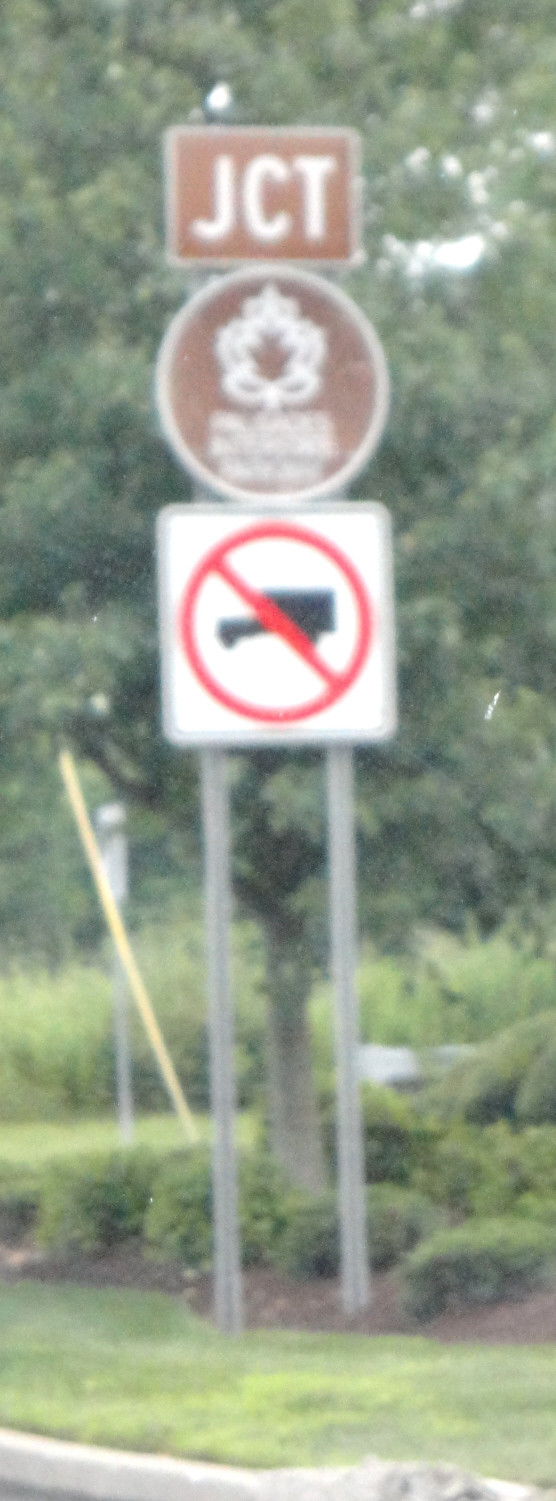This photograph, though slightly grainy, captures a detailed scene centered around a cluster of signs mounted on a silver metal pole. At the bottom of the image, the edge of a concrete curb is visible, bordered by light green and darker green grass interspersed with patches of yellowish grass. Prominently displayed are three signs: the first is white featuring a black truck circled in red with a red slash through it, indicating a "No Trucks" regulation. The second sign has a brown background with white font and a white leaf design, suggesting it might pertain to either a natural area or a specific regulation or information. The third sign also has a brown background with white font, simply stating "JCT," likely denoting a junction.

In the background, a lush, green, leafy canopy of trees is visible, along with dense green bushes and sections of brown dirt. The scene is dotted with overgrown green grass. Additionally, a slender yellow object protrudes from the ground, possibly marking something specific or acting as a utility marker, alongside another unspecified sign. The overall vista is rich in detail and suggests a location blending natural elements with man-made regulations and infrastructure.